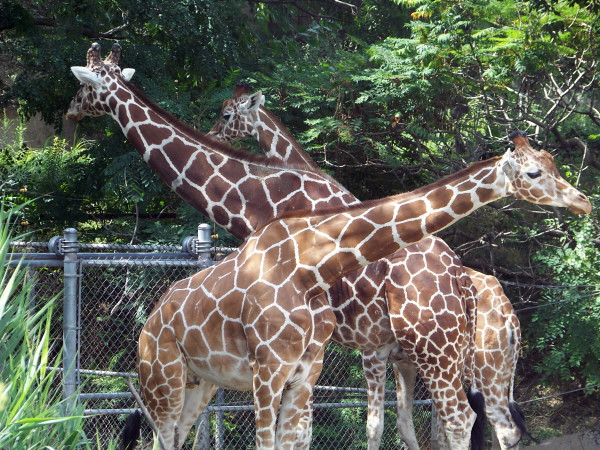This rectangular photograph, likely taken at a zoo during summer, captures three giraffes standing in an enclosure with lush, leafy greenery and a classic chain-link fence in the background. The giraffes showcase their distinct, beautiful patterns of dark chocolate brown, tile-like spots varying in hue, with yellowish-tan lines in between, gracefully covering their long necks, legs, and bodies. Two of the giraffes stand side by side, both gazing towards the left of the image, while the third giraffe in the foreground faces to the right. Their small faces, adorned with two-pointed ears and short, nubby horns, exude a serene and majestic presence. The rich, green foliage hints at the summer season, enhancing the vibrant and natural setting of these elegant creatures.